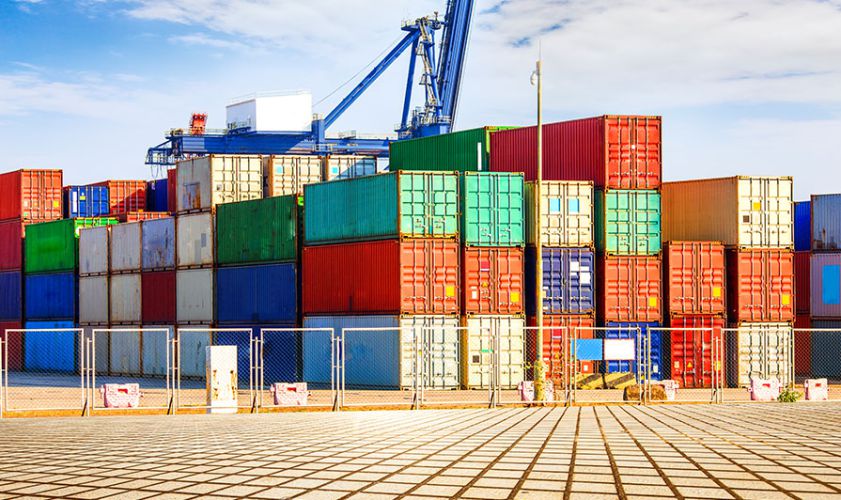The image depicts a bustling shipping yard, likely near a port, filled with a multitude of colorful intermodal containers. These large containers, which are used for transporting goods by train or ship, are stacked in varying heights, with some piles reaching up to four containers high. The containers are painted in a spectrum of colors, including white, orange, blue, green, turquoise, and red. In the background, a large blue crane can be seen, seemingly tasked with the loading and unloading of these containers, indicating a highly active industrial area.

A prominent chain-link fence cordons off the container area, reinforcing the sense of an organized and secure storage environment. In the foreground, there is a surface that looks like tiled concrete, providing a solid base for vehicles or pedestrians navigating the area. The sky above is mostly cloudy with patches of blue, suggesting a day with mixed weather conditions. The overall scene captures the busy, industrious nature of port activity in an outdoor setting.